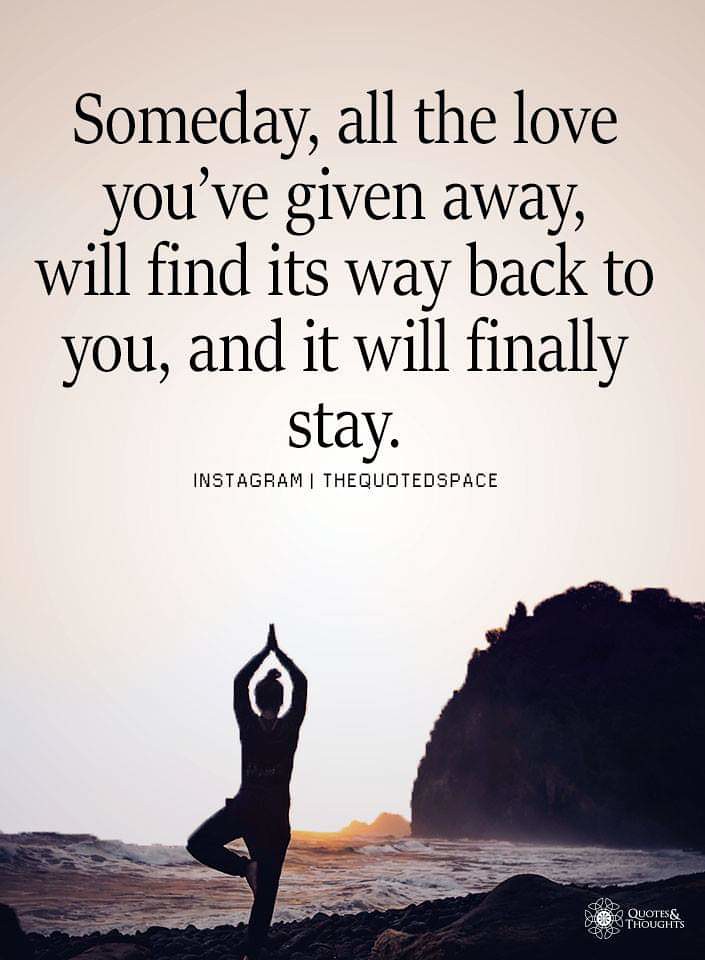The image is a color photograph in portrait orientation, depicting a serene beach scene at sunset. The sky above is a pale, cloudy white, blending into the horizon where the sun sets in the distance, casting a gentle glow. In the foreground, slightly to the left of center, stands the silhouetted figure of a woman gracefully performing a yoga pose with her arms raised, palms pressed together, and her left foot resting against her right leg. Behind her, ocean waves crash onto the shoreline which is visible in the lower right corner, emphasizing the high tide. To the right of the woman, a large, rounded hill or stone cliff rises in silhouette. 

At the top of the image, in bold black text, is an inspirational quote: "Someday, all the love you've given away will find its way back to you and it will finally stay." Below this, in smaller black text, is the source: "Instagram, the quoted space." At the bottom right corner, there is a white circular logo next to the text "quotes and thoughts." This poster beautifully combines elements of photographic realism with graphic design to convey a motivational message.